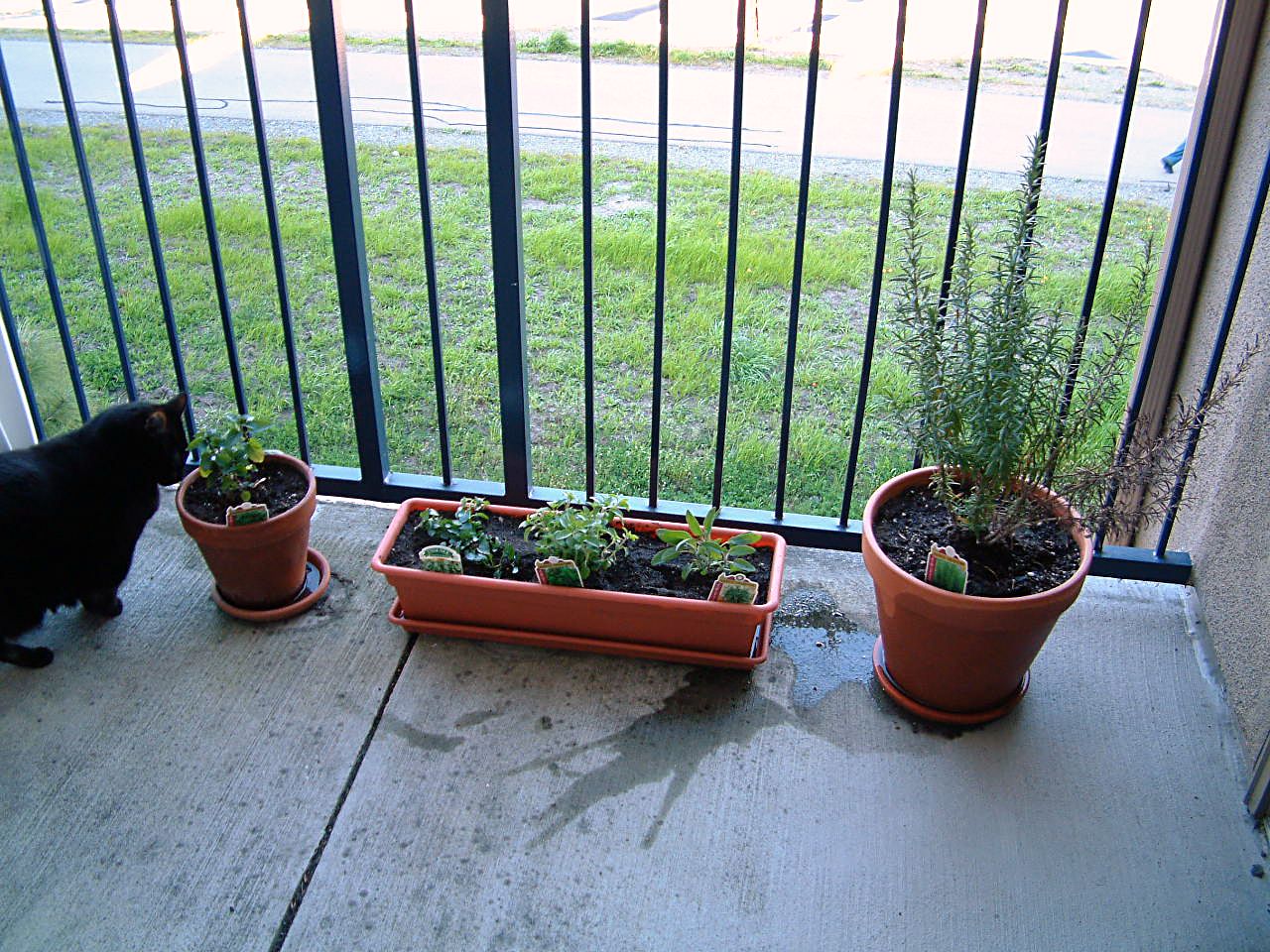The image showcases a secluded patio or backyard area with a stone floor. The space is enclosed by black iron bars, providing a view of a lush green lawn beyond the gate. There's a sidewalk visible and possibly the hint of a river in the background. In the foreground, several potted plants are arranged in a row. These plants are housed in brown and red clay pots of varying shapes and sizes. The leftmost plant sits in a round pot with a red base and a green plant sprouting from it. The center planter is rectangular and contains several small herb-like plants, each adorned with tags. To the right is another round pot, larger than the first, containing a solitary plant with fine needles. Nestled beside these pots is a curious black cat, sniffing at one of the plants. Adjacent to the potted plants, a sliding glass door might be partially visible. The overall scene is tranquil, blending elements of nature with domestic life.